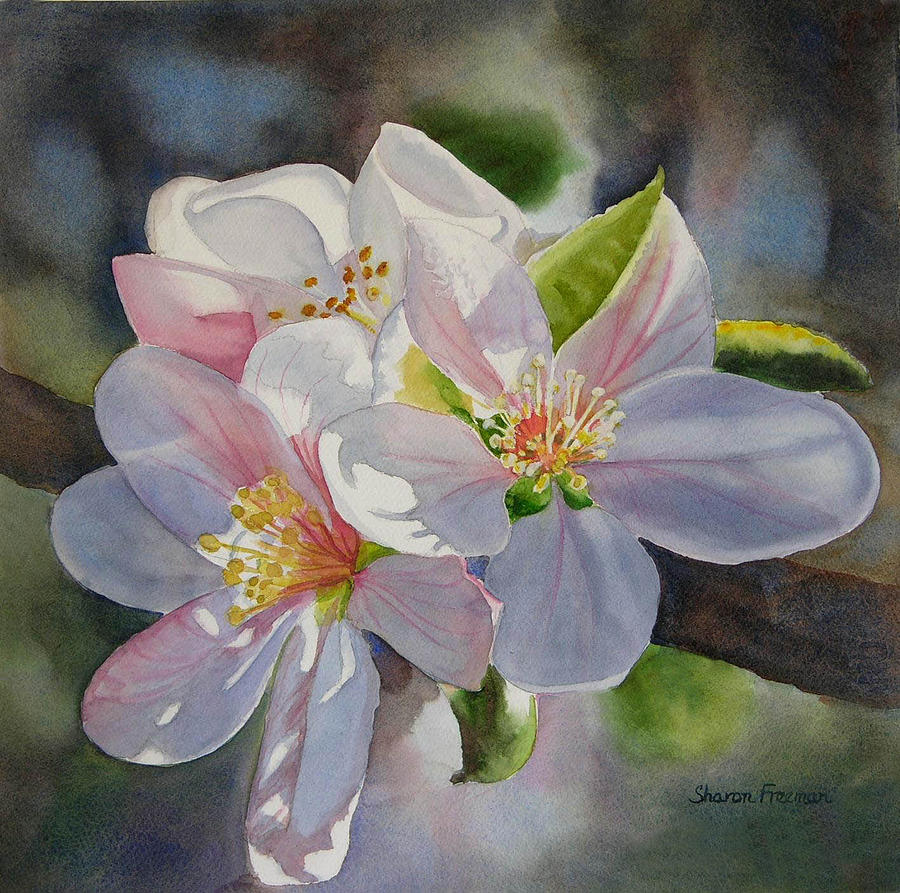This detailed watercolor painting by Sharon Freeman, signed in the bottom right-hand corner, features an up-close depiction of vibrant flowers emerging from a thick, sturdy brown branch. The three prominent flowers, open wide and varied in petal count, showcase a stunning mix of lavender, dark purple, bright pink, and white hues, with vibrant yellow stamens and intricate pink stems accentuating their centers. The surrounding backdrop is a blend of dark, muted colors, with subtle greens and blues that create a blurred effect, drawing attention to the detailed and elaborate floral arrangement in the foreground. In addition to the main flowers, there are also indistinct petals and green leaves that add depth and complexity to the composition.